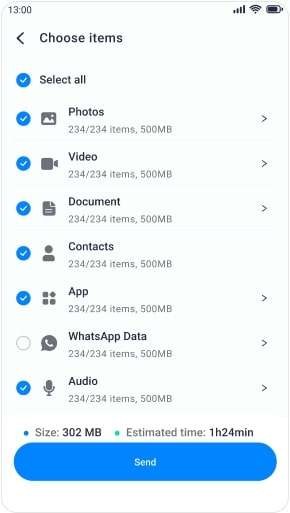The image is a screenshot of a phone's settings menu with a white background. In the top left corner, the time is displayed as 1300 in 24-hour format. On the top right corner, there are service bars, a Wi-Fi signal indicator, and a nearly full battery icon.

At the top of the menu, there is a header that reads "Choose Items" accompanied by a back button. Below this header, the following selectable items are listed in order: "Select All," "Photos," "Video," "Document," "Contacts," "App," "WhatsApp Data," and "Audio." Each item, except "WhatsApp Data," has a blue box with a white checkmark to its left indicating selection. To the right of each item, there are arrows that likely lead to further options, except for "Contacts," which lacks an arrow.

Each listed item has an associated icon for visual representation: a photo icon for "Photos," a video reel icon for "Video," a document icon for "Document," a contacts icon for "Contacts," a WhatsApp icon for "WhatsApp Data," and a sound wave icon for "Audio."

At the bottom of the menu, there is a large blue "Send" button. Above the "Send" button, the size of the items selected is indicated as "302 MB," with an estimated transfer time of "1 hour 24 minutes."